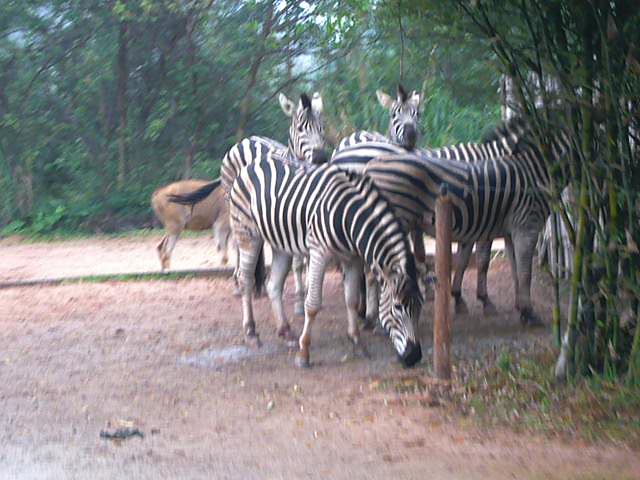In this slightly blurry color photograph, a group of five zebras stands in a clearing within a wooded area. The foreground features a zebra with its head bent down, grazing on the grass near the base of a wooden post. Two of the zebras have their heads hidden in a cluster of thin, bamboo-like trees, and are facing away from the camera. Behind these three, two more zebras can be seen; one gazes directly at the camera, while the other looks off to the right. The ground beneath them is mostly dirt with some patches of grass and a small muddy area. In the background, a large, brown, deer- or horse-like animal is partially visible, though its head is obscured. The scene is framed by a dense forest of green-leaved trees, providing a lush backdrop to the tranquil setting.